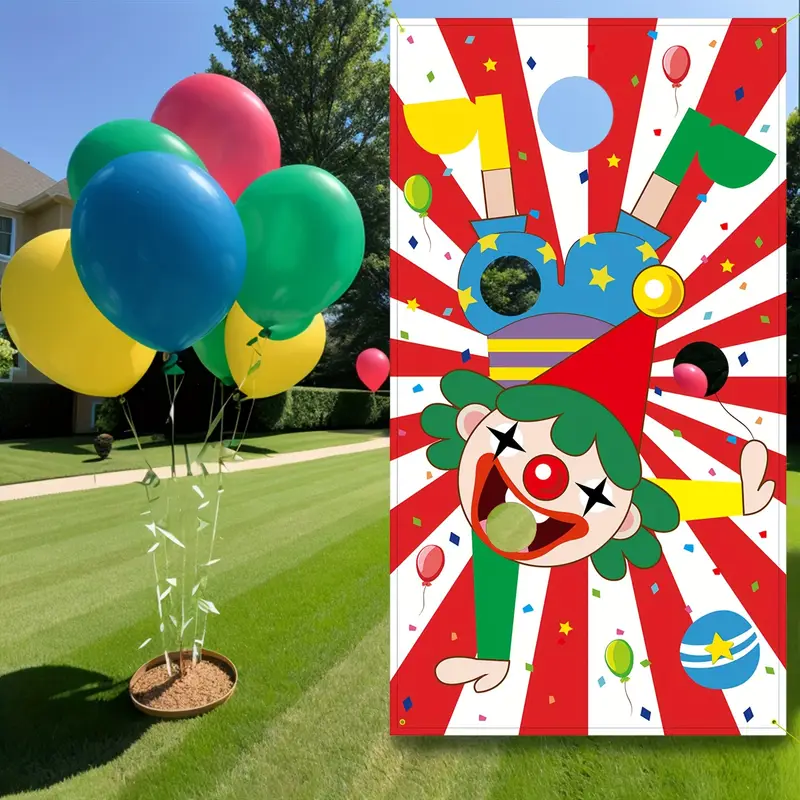In this vibrant outdoor scene set in a meticulously manicured backyard, the photograph captures a festive birthday party setup. Dominating the right side is a tall, colorful clown cutout board designed for photo opportunities, where children or adults can stick their faces through strategically placed holes. The clown is depicted in a handstand, balancing on its right hand, with its left hand pointing upwards. It features a bright, smiling face with distinctive green hair, a red and gold dunce hat, white eyes accentuated with black stars, a red nose, and a wide, red mouth. The clown's outfit includes a purple blouse with yellow stripes, blue shorts adorned with yellow stars, one yellow boot, and one green boot. The backdrop of the cutout board is boldly decorated with alternating red and white stripes, multi-colored stars, and an array of balloons, creating an eye-catching and jubilant atmosphere.

To the left of the cutout, a cluster of helium balloons in a mix of colors—three green, two yellow, one blue, and one red—is grounded in a small patch of soil, accentuated with ribbon-like strings. The freshly mowed grass displays neat mower lines, indicating careful lawn maintenance. In the background, the well-kept yard continues with additional grassy areas, green hedges, and a tall tree. Part of a two-story tan house with several windows is visible, enhancing the homely setting. The scene vividly conveys the joy and excitement of a celebratory gathering in a charming suburban backyard.